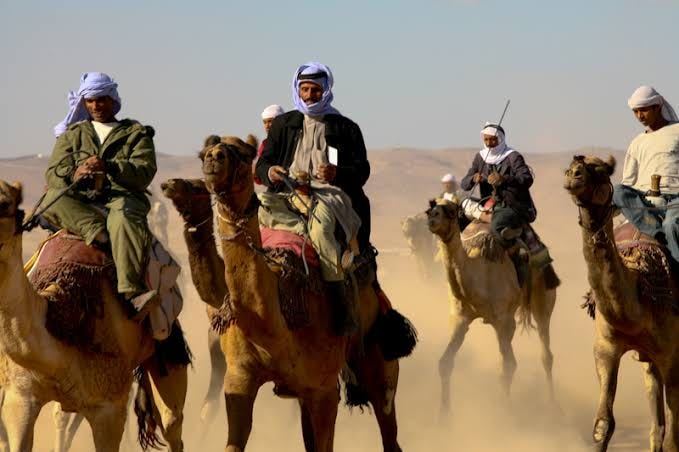This photograph captures a dynamic scene from the Middle East, where six men are traversing a desert landscape on seven camels. The men, dressed in traditional Middle Eastern attire, don turbans and loose, flowing robes that signify the region's style. Their garments include green jumpsuits, flowy shirts, pants, and black overcoats, with notable lavender turbans on two individuals. The group is moving from right to left, amidst kicked-up desert dust that partially obscures the hills in the background. The camels are outfitted with red saddlebag-like decorations reminiscent of Persian carpets. Among the riders, a couple of men on the right sport mustaches, and one appears to be younger than the rest. Hues of green and tan dominate the scene, adding to the earthy and authentic Middle Eastern ambiance of the adventure.